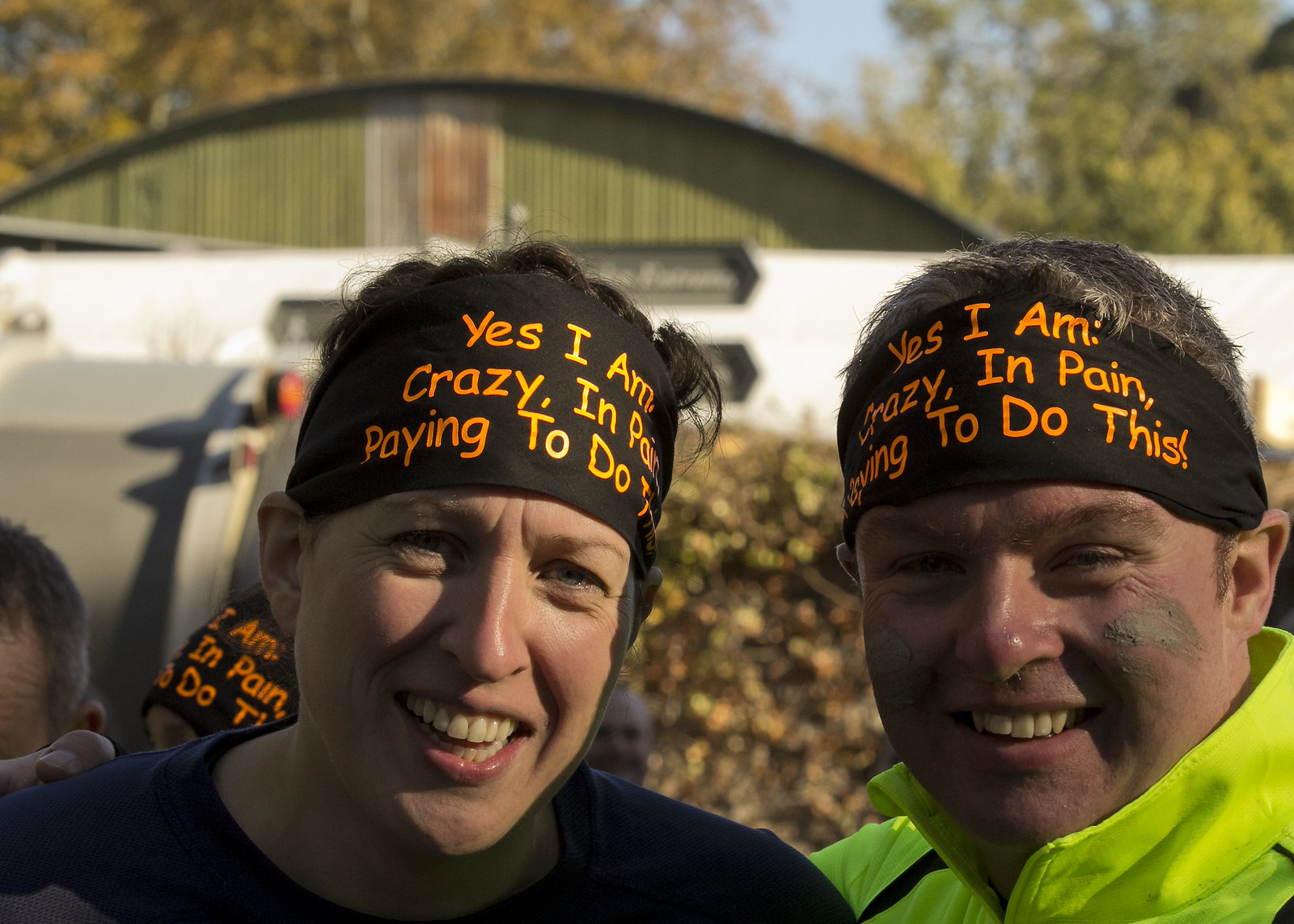In the photograph taken outside on a sunny day, two people—appearing to be a woman on the left and a man on the right—are prominently featured, both smiling with visible teeth. They’re wearing black headbands with orange letters that read, "Yes, I am crazy, in pain, paying to do this." The woman is dressed in either a dark blue or black shirt, while the man sports a green jacket. The man's face is smeared with mud, suggesting they are engaged in some sort of strenuous outdoor activity. Another person in the background can be seen wearing the same headband. The setting includes a blurred backdrop of a building, possibly a Quonset hut, with trees and a glimpse of blue sky also visible.